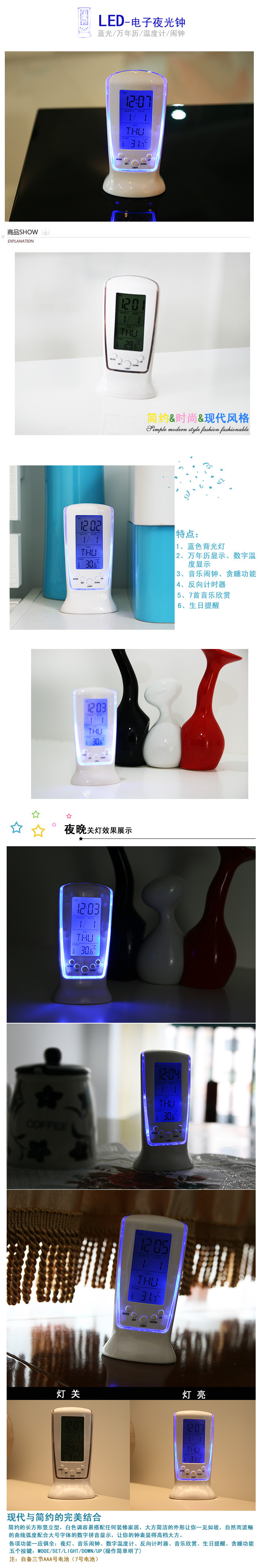The image is a vertical strip consisting of numerous smaller, thumbnail images showcasing a countertop-sitting, plastic LED device. This device, characterized by its white frame and circular base, features a blue screen, and is possibly a modern, electronic gadget such as a baby monitor or another LED-backlit item. The presentation includes several configurations: some images depict the device fully illuminated, while others show it turned off. The LED screen often presents black lines, although the text remains too small and detailed to precisely decipher. The text at the top, predominantly in small Japanese traditional characters, clearly spells out "LED" in capital letters. The device appears in various home settings — one instance places it beside a teapot, suggesting its versatile use within domestic environments. Another thumbnail shows the gadget set among vases, emphasizing its aesthetic placement. Despite a tiny list of apparent features present in one image, the detailed functionalities are not readable.